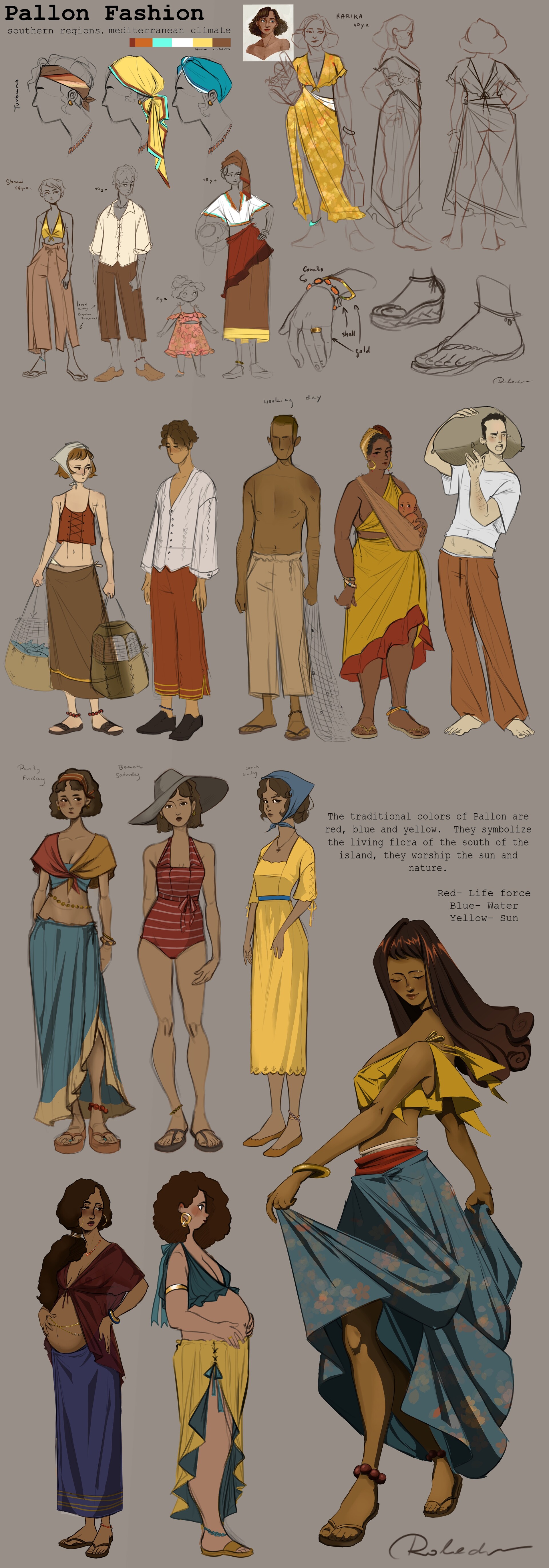The image is a tall, rectangular poster titled "Fallon Fashion," featuring a series of detailed drawings of women in various outfits, set against a gray or drab brown background. The composition consists of about five rows, each showcasing a range of fashion styles, predominantly suitable for a tropical or Mediterranean climate, with a consistent theme of loosely fitting clothes and sandals. 

At the very top, the poster showcases women adorned in distinctive headwear: a woman with an elaborate headdress and three others with headscarves in red, yellow, and blue. Below them appears a woman wearing a traditional African dress with a midriff top and a slit skirt, alongside two monochrome sketches of women.

The second row features a variety of casual and workwear: a woman in black pants just above the knee paired with a sports bra; another in a white jacket with red pants and brown shoes; a girl in a little red dress; and a woman in a red and brown skirt with yellow trim, a white top, and images of hands and feet sprinkled around.

In the third row, diverse styles continue with a white woman in a tank top and a long brown skirt carrying two bags, a figure in a white shirt with red pants and black shoes, a shirtless black man in brown pants, a black woman in a sleeveless dress, and a man, barefoot in orange pants, carrying a rock or melon.

The fourth row shows a woman in a brown dress with short sleeves, a blue skirt, and sandals; another in a frothy sun hat, wearing a red swimsuit and sandals; and a black woman in a yellow dress to her calves with a brown headscarf.

The final row features a woman with a shawl and a long blue skirt, alongside a pregnant woman in a yellow and blue skirt with a slit, wearing a sports bra. In the bottom right, a larger illustration depicts a black woman wearing a sleeveless yellow top and a blue skirt, dancing and holding her skirt to reveal her legs, signed with the name "R-O-L-A-D." Additionally, a small, unclear paragraph appears two-thirds down the image, with some visible letters like "T-H-E."

Overall, the poster illustrates around 20 different outfits, including elegant dresses, casual wear, beach attire, and worker clothes, reflecting a colorful and versatile collection designed for warm climates.